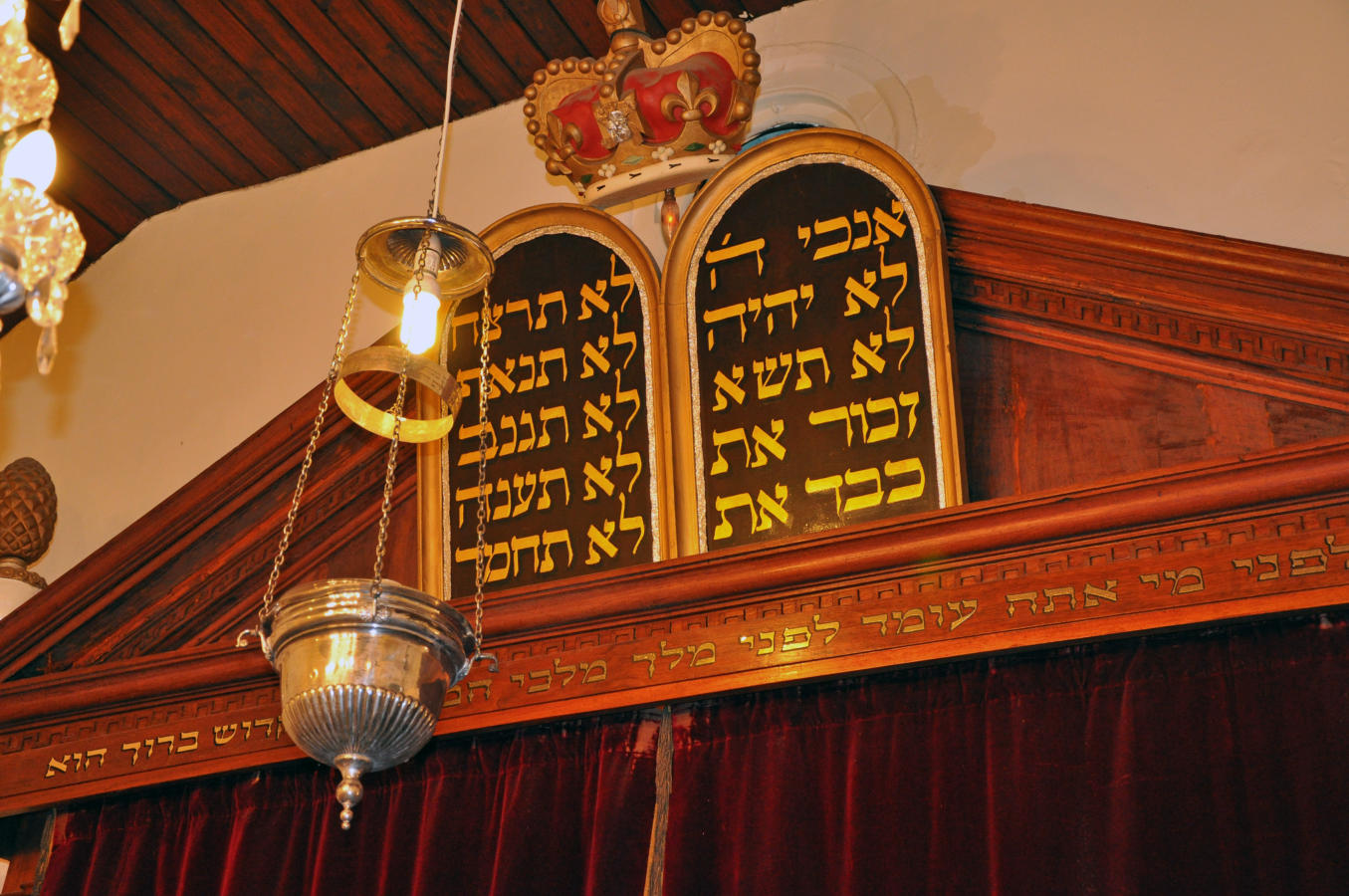This photograph captures a richly detailed, close-up view of the upper section of a sanctuary within a Jewish temple or synagogue. The indoor setting is characterized by a high-ceilinged room with a white-painted wall and a ceiling comprised of wooden planks. The focal point is an ornate triangular pediment, designed with dark wooden trim and adorned with intricate carvings.

At the center of this triangular structure are two arch-shaped tablets, featuring gold Hebrew inscriptions set against a dark brown background. Nestled between these tablets is a gold and red crown, adding to the regal and sacred atmosphere. Suspended in front of the tablets is a silver lamp, hanging by a chain with a visible light bulb beneath its lampshade.

Below the tablets, a horizontal beam also displays Hebrew writing in gold, and beneath this are rich red velvet curtains. The triangular pediment inclines from the bottom left toward the top middle of the image, creating a dynamic visual ascent. An outline of another lamp is faintly visible in the top right corner, maintaining the room's cohesive aesthetic.